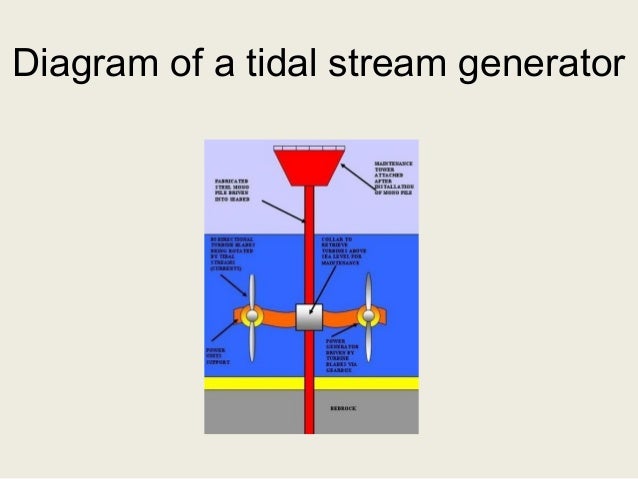The image is a detailed infographic that illustrates a tidal stream generator. The heading at the top of the infographic, set in black text on a light gray background, reads "Diagram of a Tidal Stream Generator." The central image, drawn in a portrait orientation, depicts the generator with a red conical top piece feeding into a vertical red tube. Midway down the tube, there is a silver junction box, from which orange arms extend horizontally, each supporting a white propeller or turbine on either side. The background of the diagram features an aqua blue section representing water, followed by gradient stripes of purple and yellow. At the bottom, a yellow line sits above a gray foundation layer that likely signifies bedrock. The diagram also includes numerous black text labels and arrows pointing to different components, although they are too small to be legible in this image.